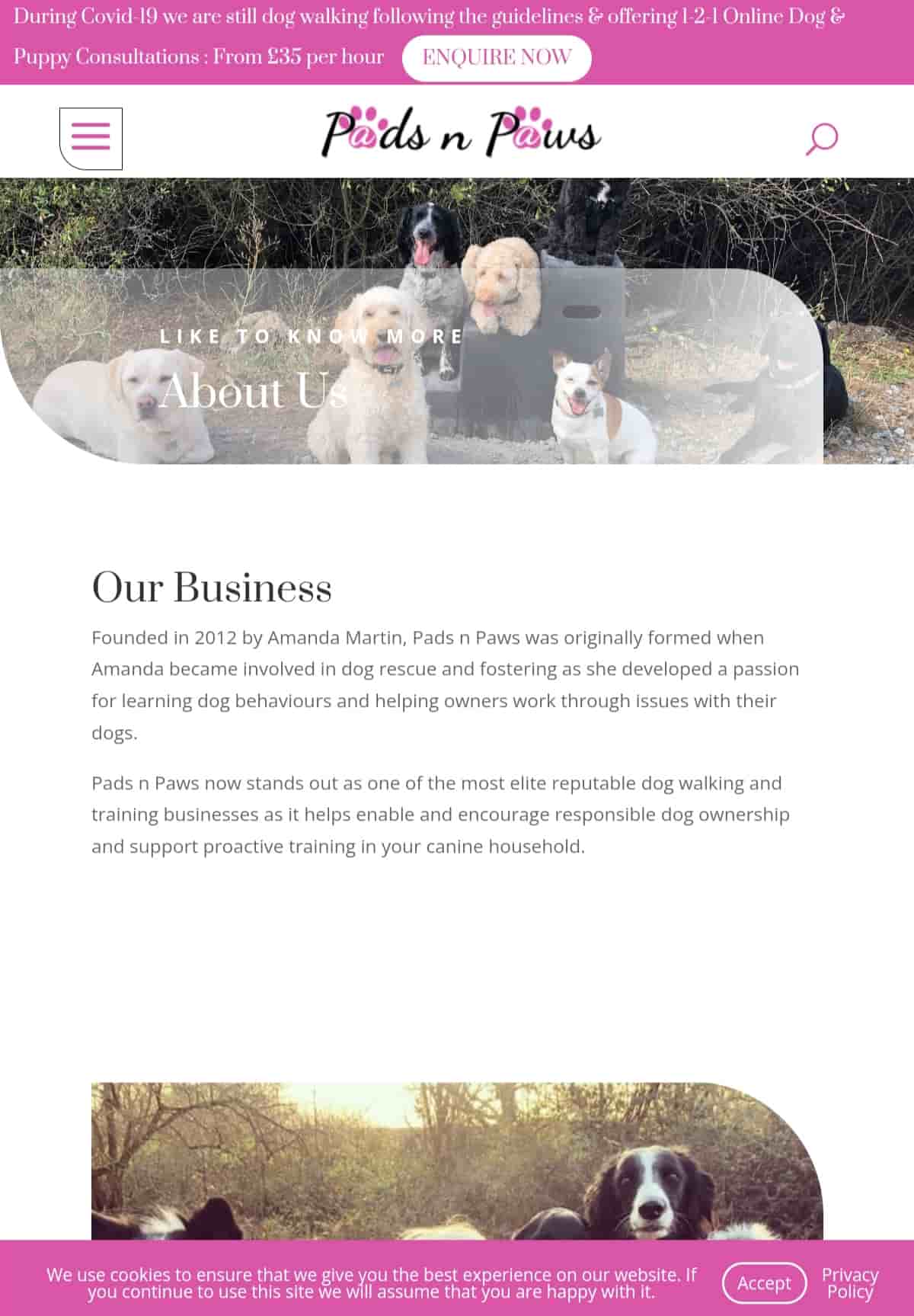The image showcased is a promotional page from a website or app, featuring a tall, vertical layout that is approximately twice as high as it is wide. 

Starting at the top, a horizontal pink banner takes up about the top 5-10% of the page. This banner contains white text which reads, "During COVID-19, we are still dog walking, following the guidelines and offering one-to-one online dog and puppy consultations from $35 per hour." To the right of this text is a prominent white button with pink text stating "INQUIRE NOW" in all capital letters.

Directly below this, occupying about another 10% of the page's height, is a white background header. In the upper left corner of this section are three horizontal pink lines, which indicate a menu. Just to the right of that, centered, is the logo for "Pads and Paws." The logo is crafted in cursive script, with the 'A's replaced by pink paw prints over white 'A's.

Beneath the header is a vibrant banner that takes up approximately 25% of the page's height. This banner features an image of small dogs looking directly at the camera, situated outdoors. Superimposed over this image is text that reads, "Like to know more about us."

Further down, there is a section titled "Our Business," accompanied by a descriptive paragraph.